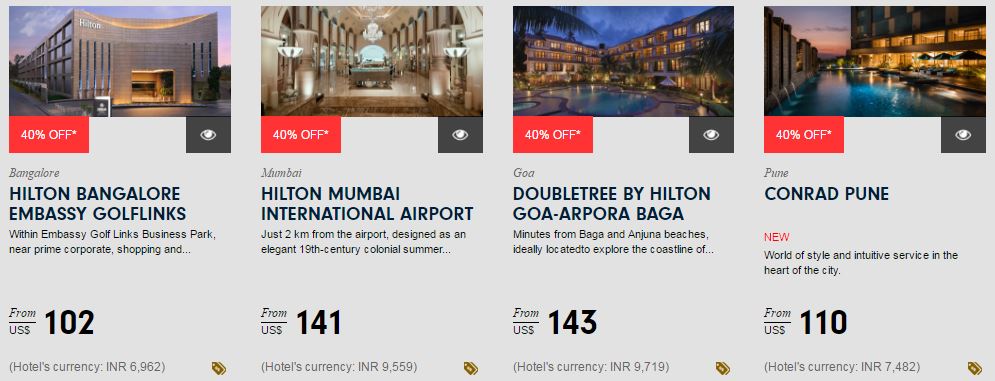This image showcases a promotional advertisement for four hotel deals, each offering a 40% discount. The advertisement is arranged in four side-by-side blocks, each featuring a different Hilton property.

1. The first block highlights the **Hilton Bangalore Embassy Golf Links**, situated within the Embassy Golf Links Business Park, proximate to prime corporate shopping areas. The top half of the block features an image of the property, while the text below notes a discounted rate of **$102**. Additionally, this block includes a "hotel currency" label.

2. The second block features the **Hilton Mumbai International Airport**, with a stylish property image at the top. The discounted rate for this hotel is listed as **$141**.

3. The third block presents the **Doubletree by Hilton Goa – Arpora – Baga**, accompanied by a vivid image of the hotel. This package is available for **$143**.

4. The fourth block showcases the **Conrad Pune**, distinguished by a "new" label. The upper section displays an inviting image of the hotel, and the special rate offered is **$110**.

Each block effectively combines visual appeal with essential pricing information, making it easy for potential guests to compare these attractive hotel deals.